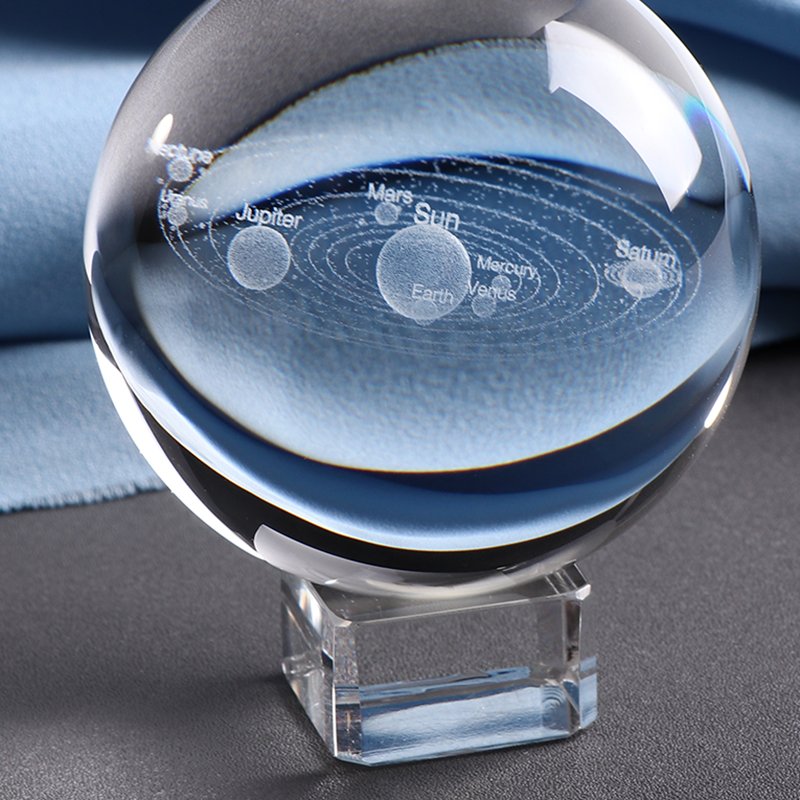The indoor daytime photograph showcases a stunning glass sphere, perched on a square-shaped glass stand, positioned on a black table. The crystal-clear orb features an intricately etched image of the solar system, displaying the Sun at the center encircled by planets labeled Mercury, Venus, Earth, Mars, Jupiter, Saturn, Uranus, and Neptune. Notably, Saturn is depicted with its iconic rings, while Earth stands out as the largest planet in this diagram. The sphere elegantly captures the orbits of the planets with circular lines radiating from the center. The glass sphere's transparency reveals a blue blanket in the background, introducing tones of lighter and darker blue into the image, contributing to a multidimensional and captivating visual effect.